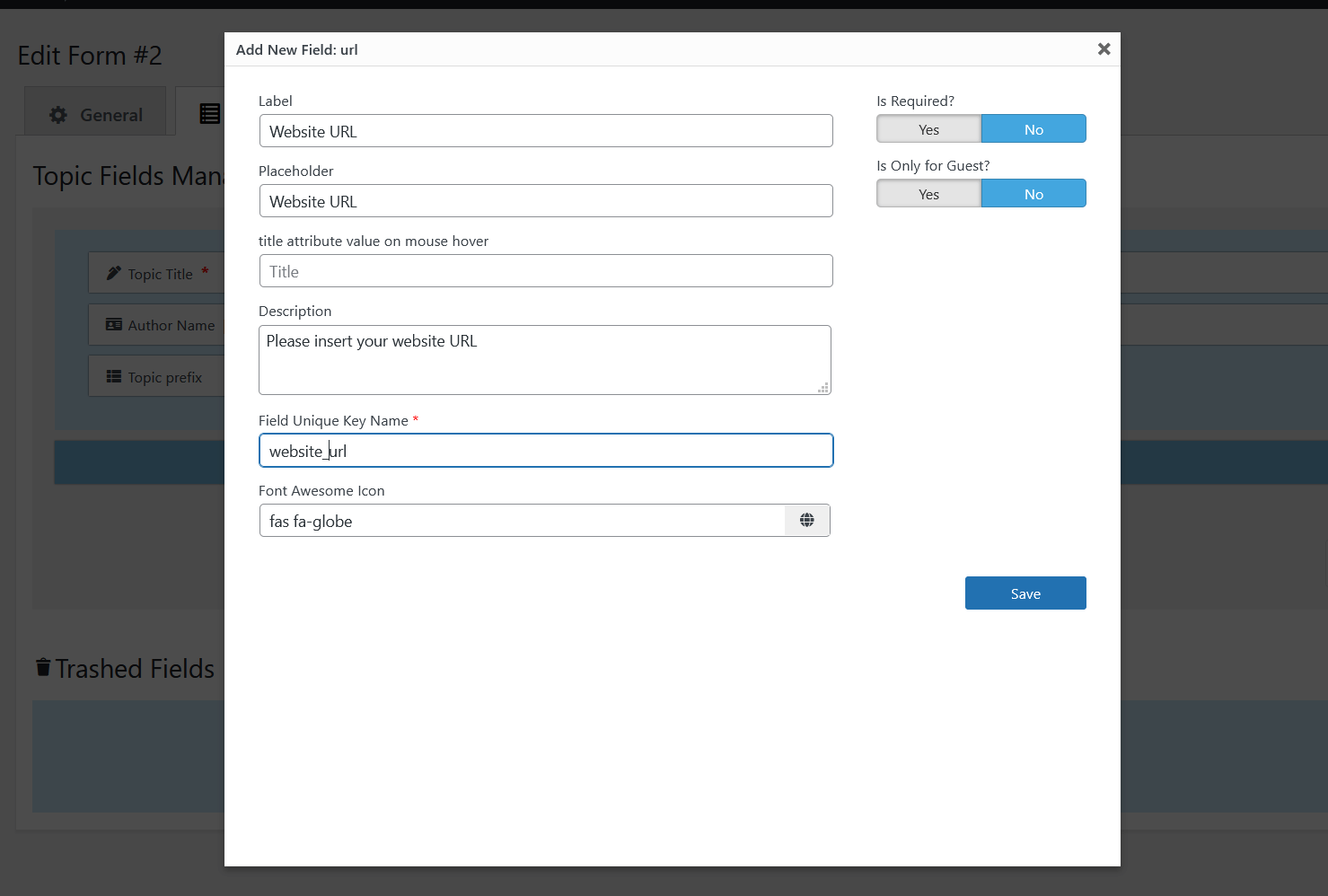The image depicts a form editor interface on a website. The main website is visible in the background but appears grayed out, likely to emphasize the active editing window. A pop-up window titled "Edit Form Number Two" is open, displaying various fields for adding a new URL. The fields include "Add New Field URL," "Placeholder Website URL," "Title," and "Attribute Value on Mouse Over." Additionally, the "Field Unique Key Name" is set to "website_URL," and there is an option to add a Font Awesome icon.

This interface seems to be part of a website-building tool, showcasing a specific step in the process of adding and configuring a new page. Users can assign a unique URL by appending custom text to the main website address. Furthermore, they can provide a name and description for this URL, and if a visitor hovers over it, a JavaScript pop-up will display the description. This detailed editor aids in creating and organizing web pages efficiently while ensuring each page has a distinct and informative URL.